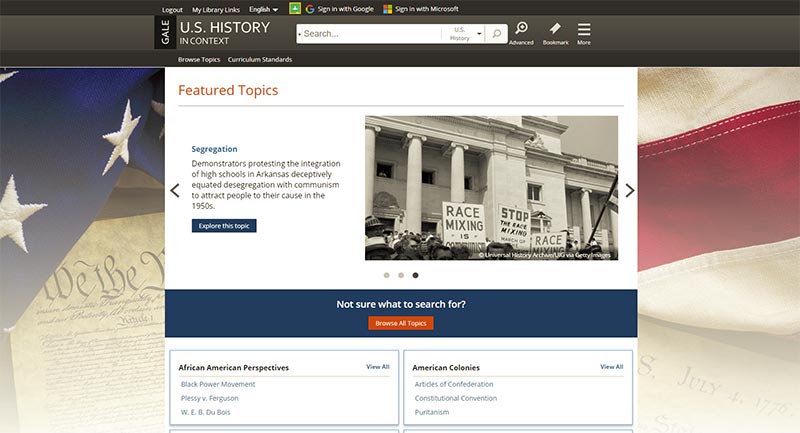The image captures a detailed view of a web page dedicated to U.S. history resources. In the background, an American flag drapes over a desk, and pages of the Constitution are faintly visible. At the top of the page, a black navigation bar features several headers, including "Log Out," "My Library," "Links," "English," "Sign in with Google," and "Sign in with Microsoft." Beneath it, a light gray bar displays the title "Gale: U.S. History in Context" alongside a search bar and a button labeled "U.S. History" with a magnifying glass icon for basic search and another magnifying glass icon for advanced search. 

Further to the right, an icon marked "Bookmark" and three horizontal bars for additional options are visible. Below these bars, a white box highlights featured topics in red text. The first topic is "Segregation," accompanied by a brief introduction and a blue "Explore the Topic" button with white text. Next to this box, there's an image of a government building with large gray columns and stone walls, in front of which people are protesting. Their signs include messages like "Stop Race Mixing. Race Mixing is Communism."

Further down, a blue text bar reads "Not Sure What to Search For?" in white text and a red button beneath it invites users to "Browse All Topics." Below this, there are two additional boxes: the one on the left highlights "African American Perspectives" and the one on the right focuses on the "American Colonies."